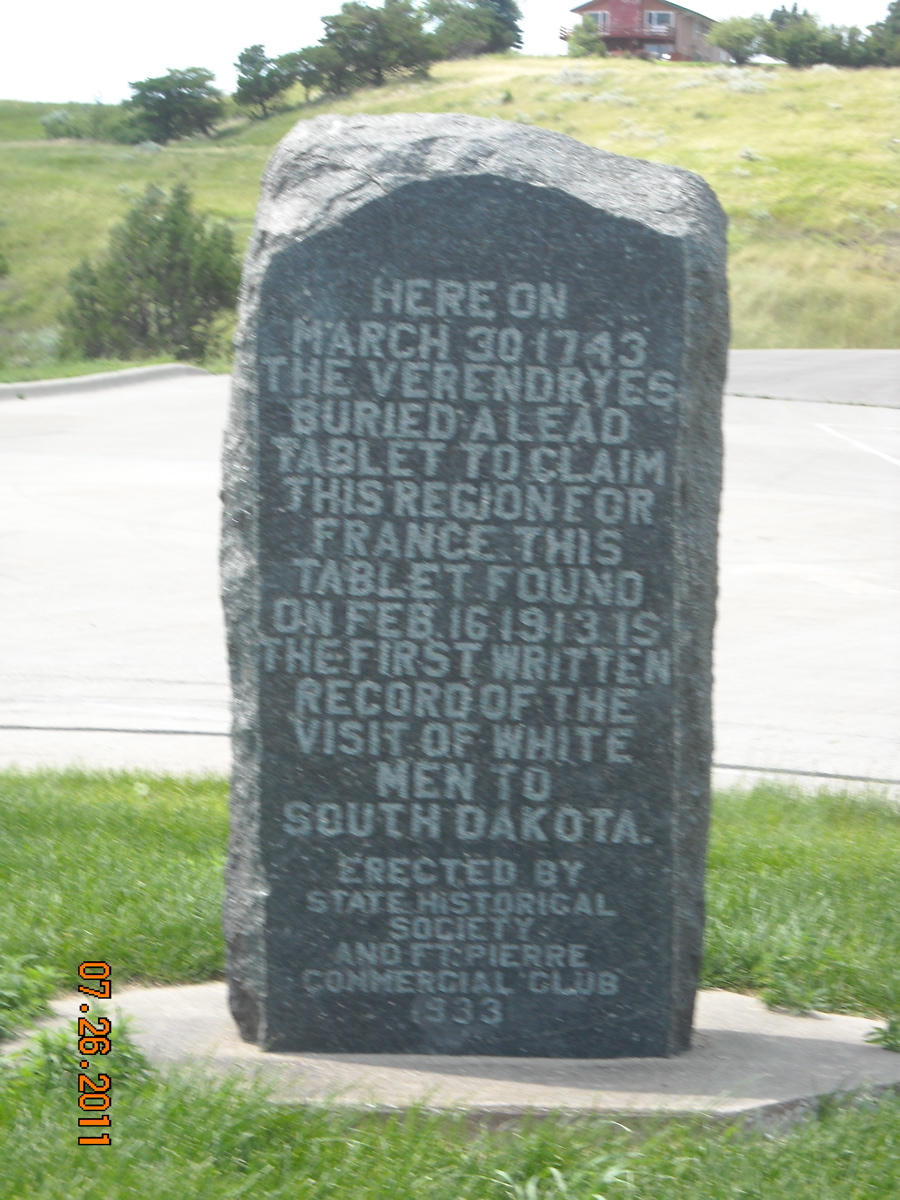This photograph depicts an outdoor scene featuring a historic stone monument that closely resembles a tombstone or headstone. Situated on a patch of grass, the monument is constructed from dark gray to black stone and rests atop a round piece of gray concrete. The stone bears an inscription that reads: "Here, on March 30th, 1743, the Varangians buried a lead tablet to claim this region for France. This tablet, found on February 16th, 1913, is the first written record of the visit of white men to South Dakota. Erected by State Historical Society and Pierre Commercial Club, 1933." The stone appears somewhat crudely formed and asymmetrical. In the background, there is a large, grassy field with a red house positioned on top of a distant hill, completing the serene yet historically significant setting.